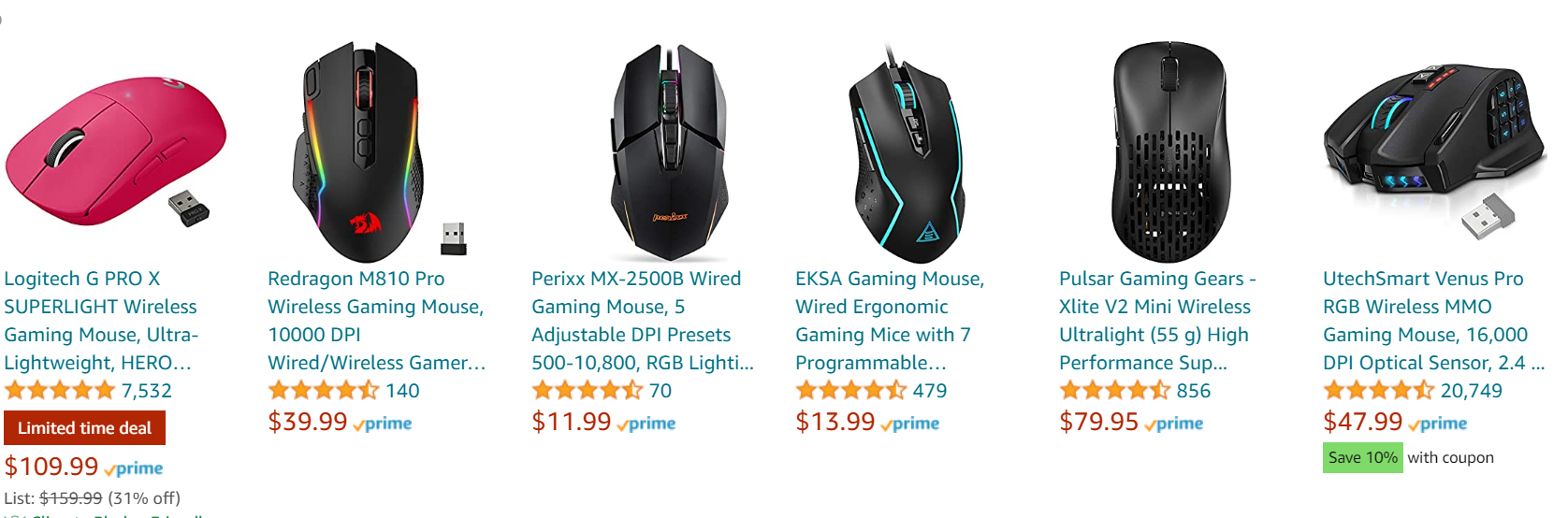This rectangular image, oriented with its longer side stretching from left to right, showcases a selection of six computer mice for sale, captured in a snapshot from Amazon. The first mouse on the left is a pastel pink wireless model labeled "Logitech G Pro X Super Light Wireless Gaming Mouse," described as an "Ultra Lightweight Hero..." in blue text. It boasts an impressive five-star rating from 7,532 reviews. Below that, a red box with white text highlights a "Limited Time Deal" priced at $109.99, with the Prime logo indicating fast shipping.

Next to it, the second mouse is black with rainbow stripes and features a red emblem at its base. It, too, is wireless. The text, also in blue, reads "Red Dragon M18 Pro Wireless Gaming Mouse" followed by "10,000 DPI Wired Gamer...". This mouse has garnered four and a half stars from 140 reviews and is priced at $39.99. Like the Logitech, this product is available for Prime shipping.